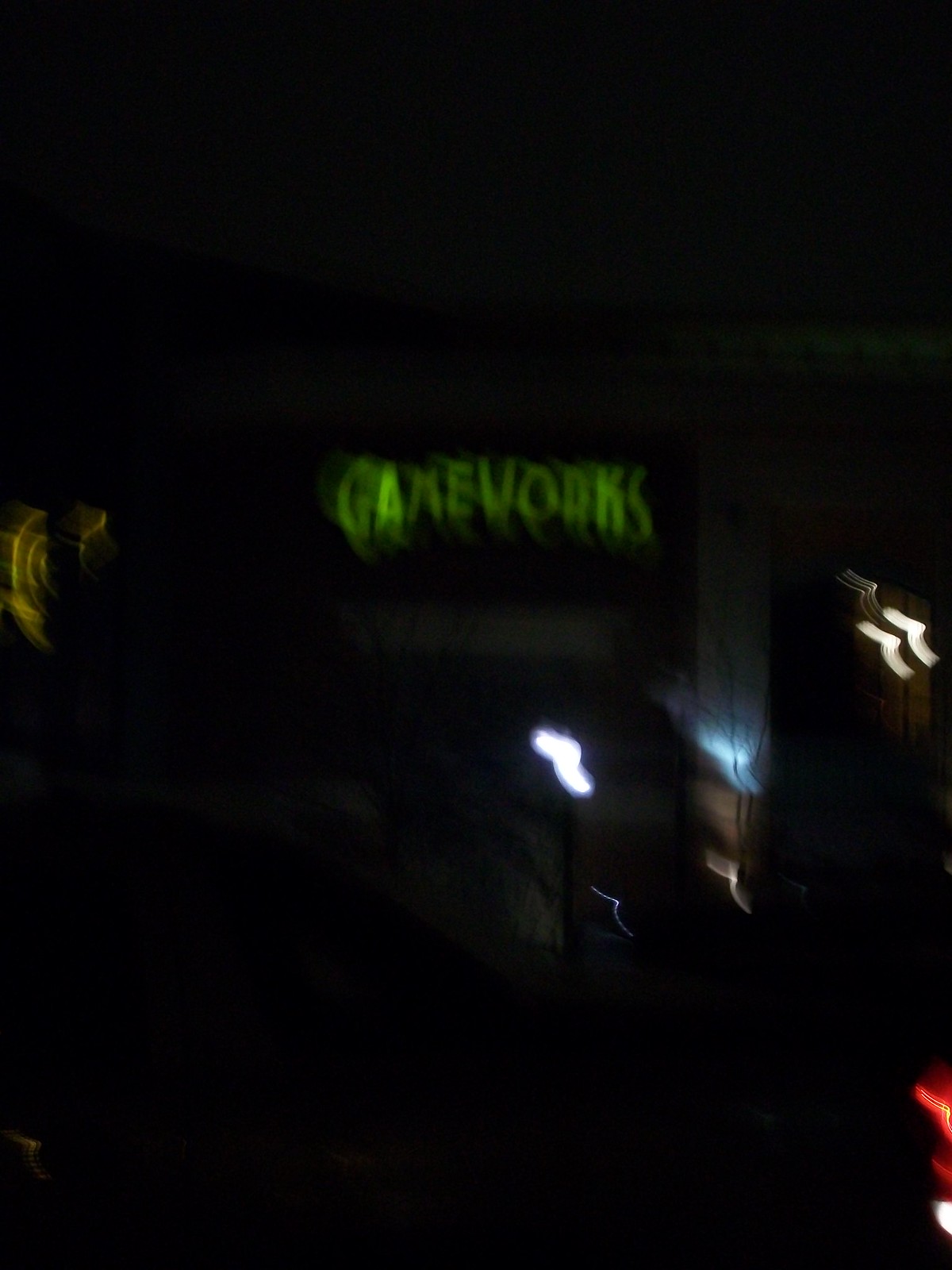The image captures a night scene, likely from across a street, and appears to be largely dark except for sporadic bursts of color and light. Dominating the scene is a blurred GameWorks sign in glowing green letters, situated on a building that seems to have a brown and gray facade. Below this sign, further enhancing the mystery of the image, are various light streaks: a red light, resembling the tip of a crayon, extends from the bottom right corner, while a nearby white light sits just beneath it. Midway up and slightly to the left, a bluish-white light emanates from a gray object, and a small white light peaks above it. To the far left edge, there's a faint, spiraling green display. Adding to the scene’s complexity, golden rings form a layered pattern below the GameWorks sign. A streetlight and possibly a car’s taillight show at the bottom, hinting the photo might have been taken from a sidewalk across the street.